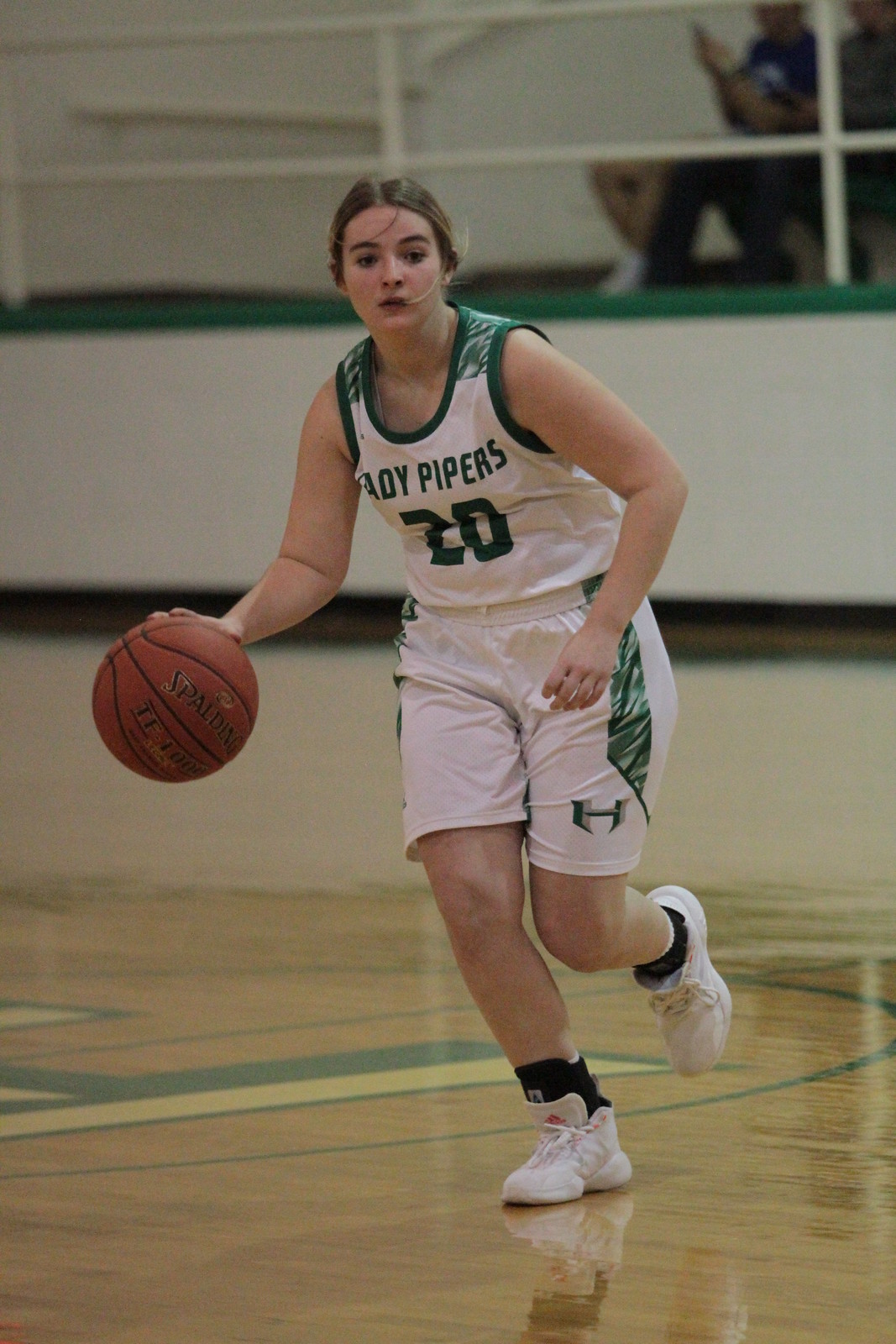This photograph vividly captures a female basketball player in motion on the court, actively dribbling the ball with focused determination. She is wearing a white uniform adorned with green details, including a green trim on the shoulders and the sides of her shorts. The jersey reads "Lady Pipers" with the number 20 prominently displayed. Sporting a practical hairstyle, her hair is pulled back into a bun, suggesting her readiness for the game. Her footwear consists of white sneakers complemented by black socks and ankle braces. The gymnasium's wooden floor features green and yellow designs that echo the team's colors. In the slightly blurred background, the bleachers and a couple of indistinct spectators are visible, enhancing the sense of an ongoing game. The overall scene captures the dynamic energy of the player and the atmosphere of the basketball court.